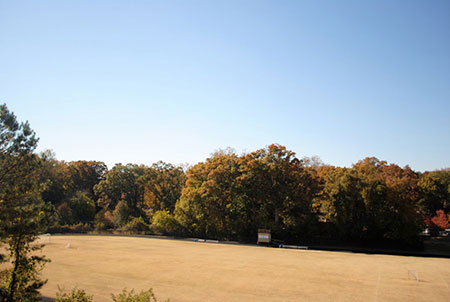This outdoor photograph, taken on a sunny day with a cloudless, vibrant blue sky, captures a serene, expansive scene blending woodland and field. The background consists of a dense forest with trees predominantly green, interspersed with hints of red, orange, and yellow, suggesting early fall. The treetops are just beginning to turn, adding a touch of seasonal transition. The foreground features a well-worn field, possibly a soccer field, with sun-bleached grass tinted brownish-green from extensive use and exposure to sunlight. On the left side of the foreground, there is a section of green trees providing a splash of verdant color. Additionally, a silver object, possibly a storage unit or water tank, is visible against the forest backdrop. This modest yet detailed image captures the essence of a well-loved, rustic outdoor space transitioning towards autumn.